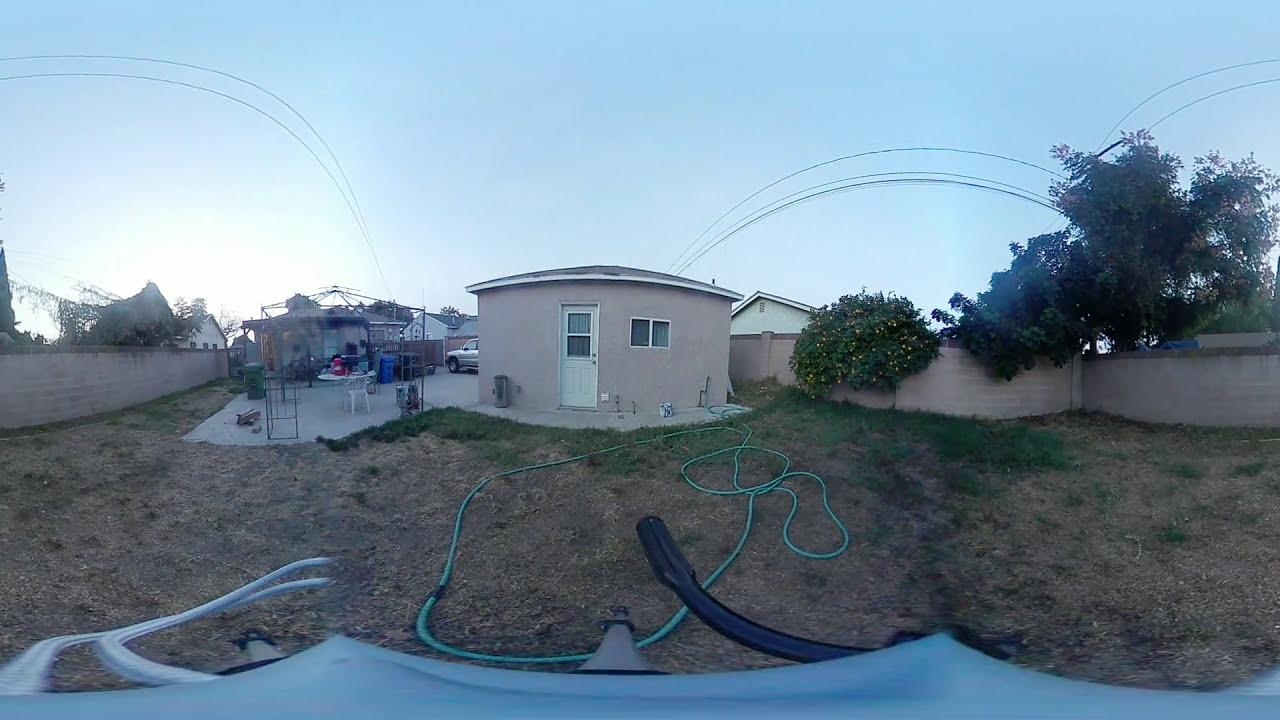The image is a color photograph showcasing a small backyard area with a house in the background. The yard itself is a mix of splotchy, patchy grass and dirt, with a long green hose lying haphazardly across it. To the left side near the back of the house, there's a white outdoor table accompanied by a couple of chairs, with a black piece extending over the table, suggesting some sort of canopy or awning. A blue trash can is also visible on the concrete area adjacent to the table, which might be part of a small back patio area.

Off to the left side of the house is a driveway area containing various items, including the table and chairs along with a parked car. Surrounding the yard is a brick fence, with trees overhanging it, including a taller tree and possibly a lemon tree bush. Utility power lines can be seen overhead against the blue sky. The overall scene is slightly distorted on the periphery, indicating it might be taken with a wide-angle lens.